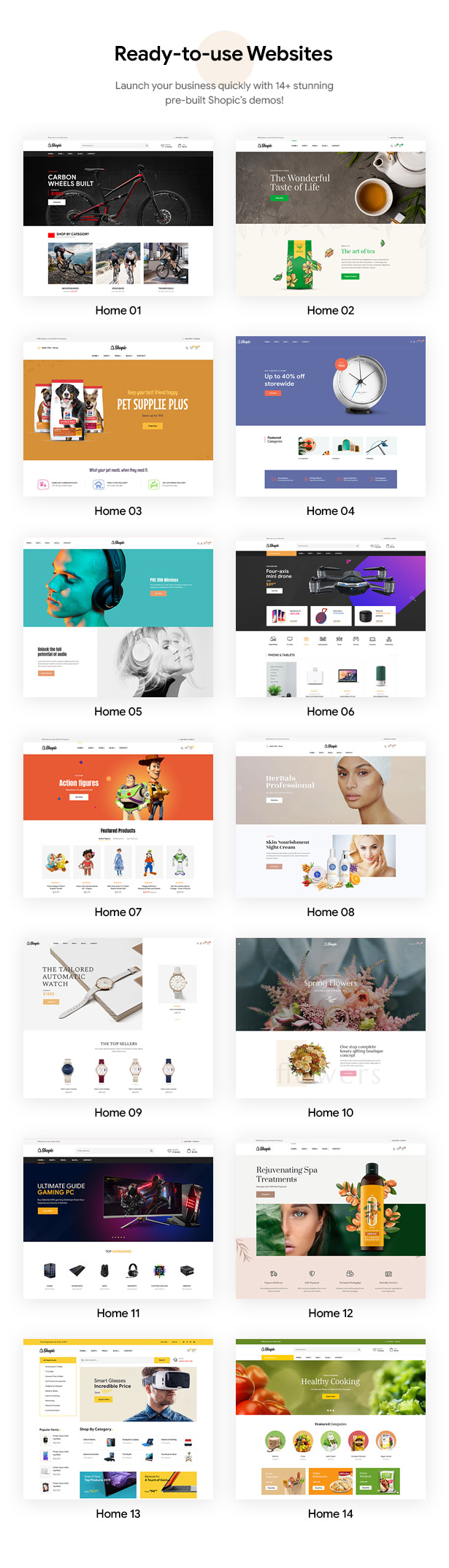This image showcases an advertisement for "Ready to Use Websites" designed to help businesses launch quickly. The display includes a collage of 18 colorful website templates, arranged in two columns with nine templates on each side. Each template features a distinct, bold color stripe across the top, in hues ranging from black and purple to aqua and orange. Despite the blurry quality making some details hard to discern, the various examples depict different types of websites catering to diverse industries. Among the notable visuals, there's a template featuring a person in a beauty turban, suggesting a wellness or beauty blog, a construction-themed site, another highlighting headphones, and one potentially featuring food, indicating a culinary focus. The vibrant array of templates emphasizes versatility, aiming to cater to a wide range of business needs.